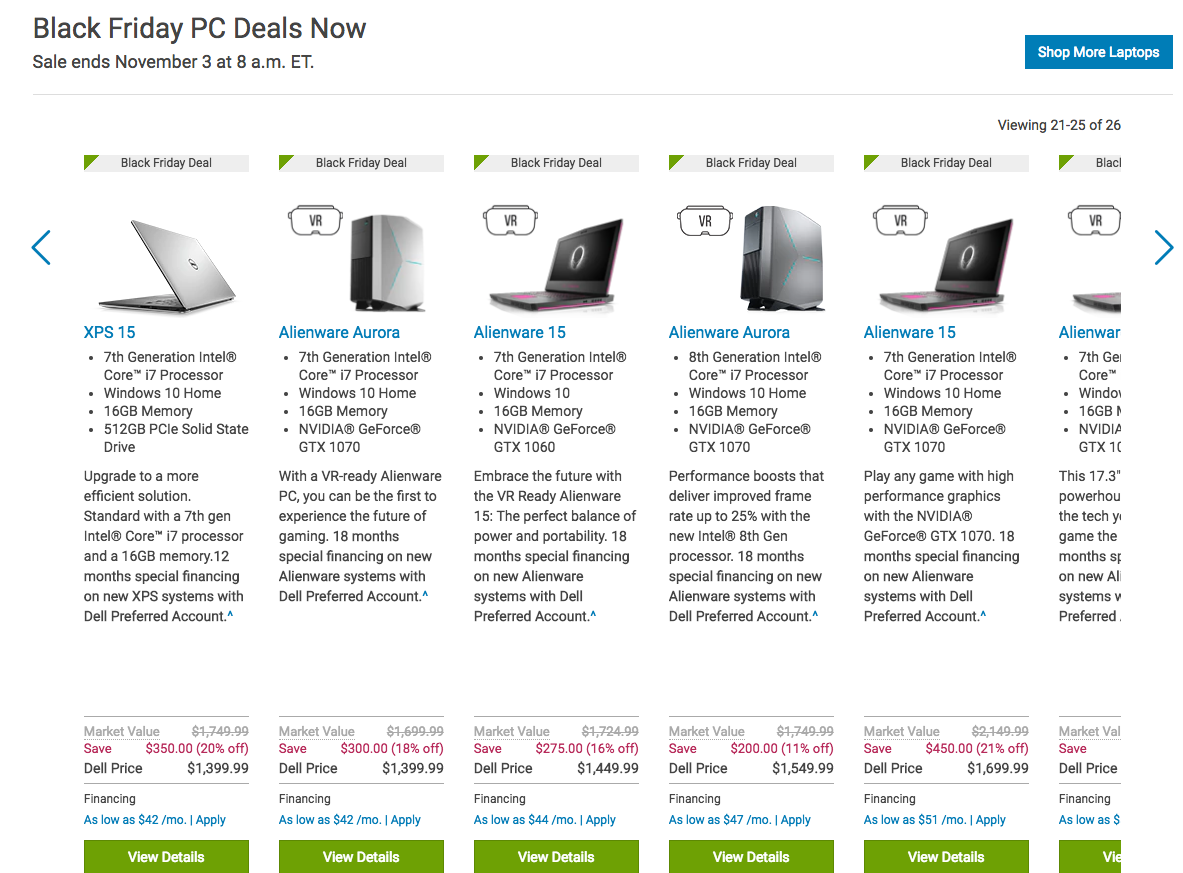The image showcases a website advertising a Black Friday sale featuring five different PC models. The sale is prominently noted to end on November 3rd at 8 a.m. ET. In the top right corner, there's a blue button with white text urging visitors to "Shop More Laptops." 

The five visible models on the screen are as follows:

1. **XPS 15 Notebook Computer**
2. **Alien Aurora Desktop** - Designed to be suitable for virtual reality.
3. **Alienware 15 Notebook** - Also suitable for virtual reality.
4. **Alienware Aurora VR** - Equipped with an 8th generation Intel processor. It offers a $200 discount, bringing the price down to $1,549.99. There's an option for financing, starting as low as $49 per month.
5. The caption also mentions a sixth model, but this is partially cut off from the view.

At the bottom of each product listing, there is a green button with white text labeled "View Details" for further information.